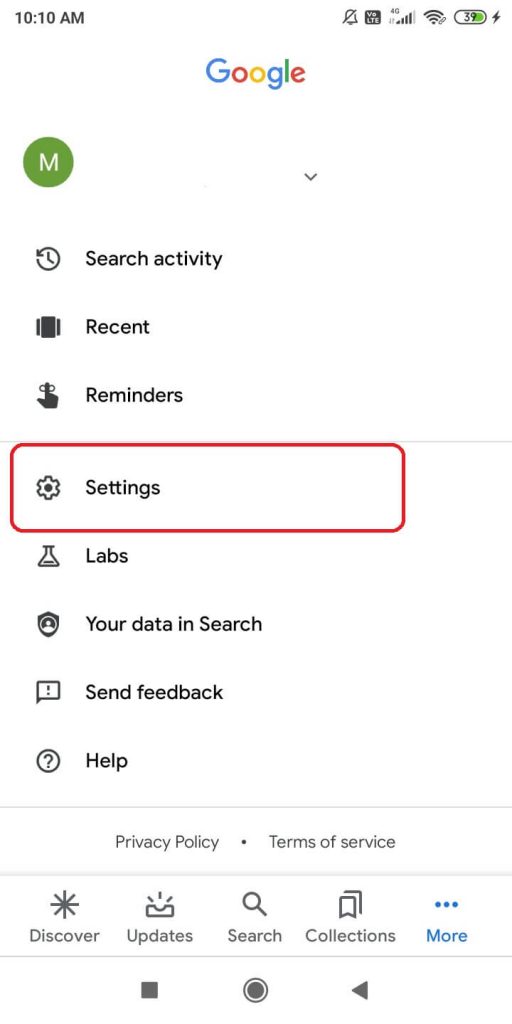Screenshot Description: 

The screenshot is of a cell phone displaying a Google interface with a black background. At the very top, there is a status bar that includes the time "10:10 a.m." on the left side, while the right side shows icons for Wi-Fi, battery, and signal strength — all in a bolded gray color. 

Below this, centered approximately two lines down, is the Google logo, spelled with a blue capital "G", red "o", yellow "o", blue "g", green "l", and red "e".

On the left-hand side of the screen, there is a green circle containing a white capital "M". Alongside this, left-aligned, is a vertical list of menu options in small, bolded black text:
- Search Activity
- Recent
- Reminders
- Settings (this option is highlighted with a red rectangle drawn around it)
- Labs
- Your Data in Search
- Send Feedback
- Help

Further below, centrally positioned between two light gray horizontal lines, is a centered decimal point. To its left in gray text is "Privacy Policy," and to its right, "Terms of Service."

At the bottom, there is a row of icons with corresponding labels:
- Discover
- Updates
- Search
- Collections
- More (highlighted in blue with three horizontal dots above it)